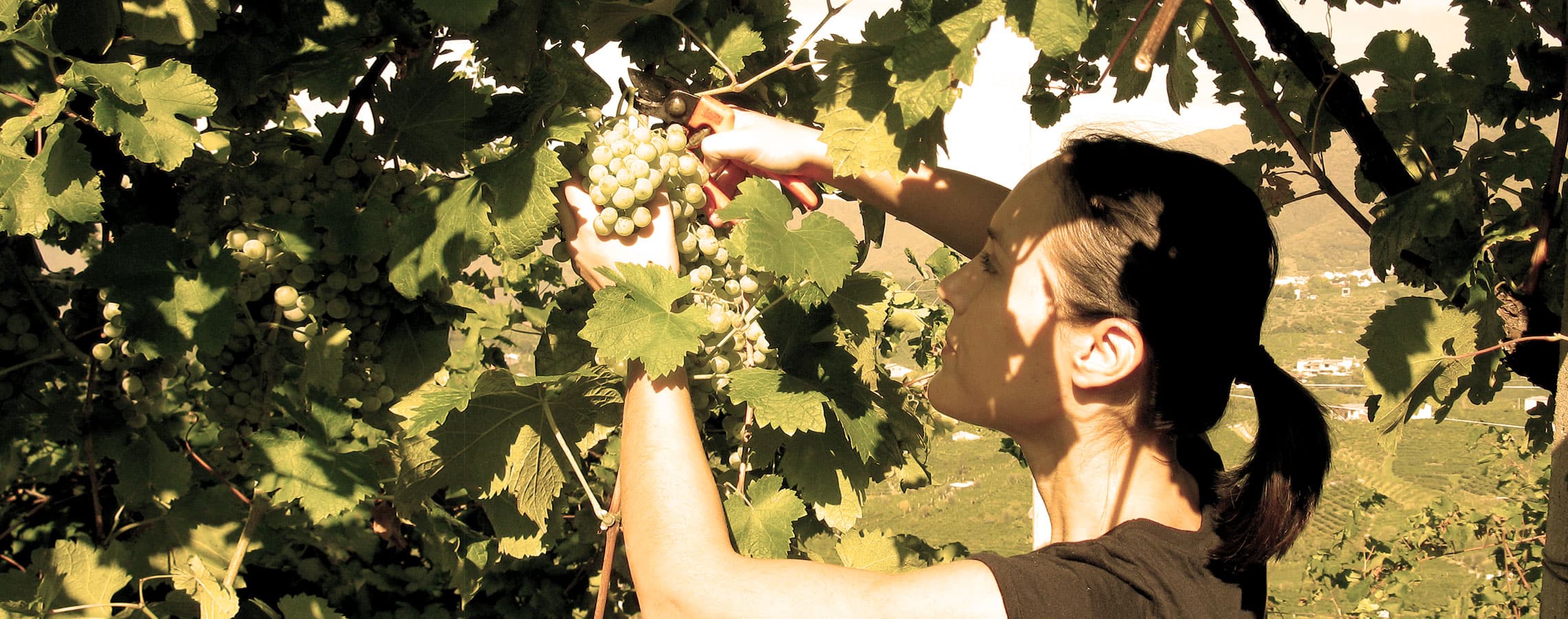In this image, a Caucasian woman with dark hair tied back in a ponytail is depicted picking green grapes from a lush grapevine. The vignette is bathed in soft sunlight, which illuminates her hands and casts a warm glow on her ears. She is dressed in a short-sleeved gray t-shirt and is focused intently on the green grapes she delicately plucks. Surrounding her are vibrant green leaves from the grapevine, forming a natural canopy. Below, a verdant valley stretches out, dotted with sporadic white structures that might be buildings, albeit faint and partially obscured. The sky in the background has a grayish hue, adding a subtle contrast to the scene. The serene agricultural landscape and the woman's attentive demeanor capture a moment of quiet labor and connection with nature.